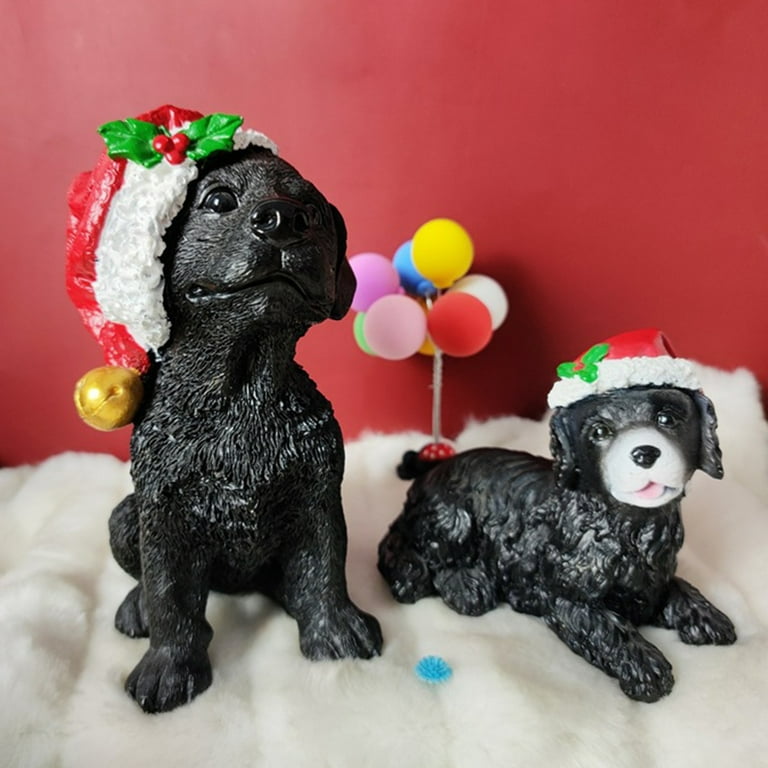In this festive holiday scene, two charming black dog sculptures, made from a shiny, rubbery material, are set against a striking solid red background. The ground is covered in fluffy white cotton, simulating a snowy landscape. The dogs, both adorned with Santa hats featuring a white fur brim, holly leaves, and one hat with a big gold bell on the end, are situated amidst this wintry setting. The dog on the right sits happily with its tongue playfully sticking out, while the dog on the left has a more neutral expression, gazing upwards with a white snout and black nose. Both dogs are complemented by a backdrop of colorful fake balloons, affixed to metal rods and a red circular base with white polka dots. A blue flower also rests on the snow between the dogs, adding an extra touch of detail to this whimsical holiday tableau.